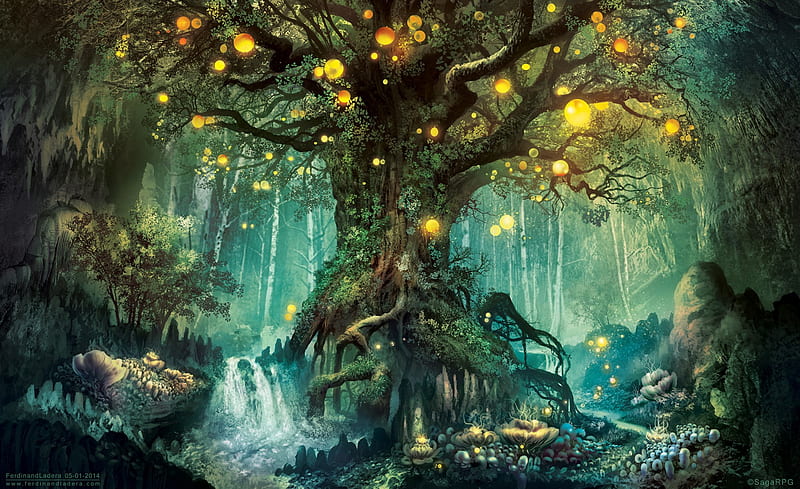In this mesmerizing fantasy painting, a colossal tree dominates the center, its grand stature adorned with vibrant green moss and thick roots sprawling outward from its base. The tree's branches extend skyward, interspersed with glowing yellow and orange orbs of various sizes, casting an ethereal light across the scene. A gentle waterfall cascades down on the left, collecting in a tranquil water area surrounded by small plants, mushrooms, and vibrant greenery. The backdrop reveals a dense array of white birch trees, their pale trunks forming a stark contrast against the dark, shadowy edges of the painting. The composition is completed with rocky outcrops and additional, smaller waterfalls, creating the sense of an enchanting, illuminated grove shrouded in mystery. The bottom of the image includes a small copyright mark for “Saga RPG," hinting at a fantastical narrative.